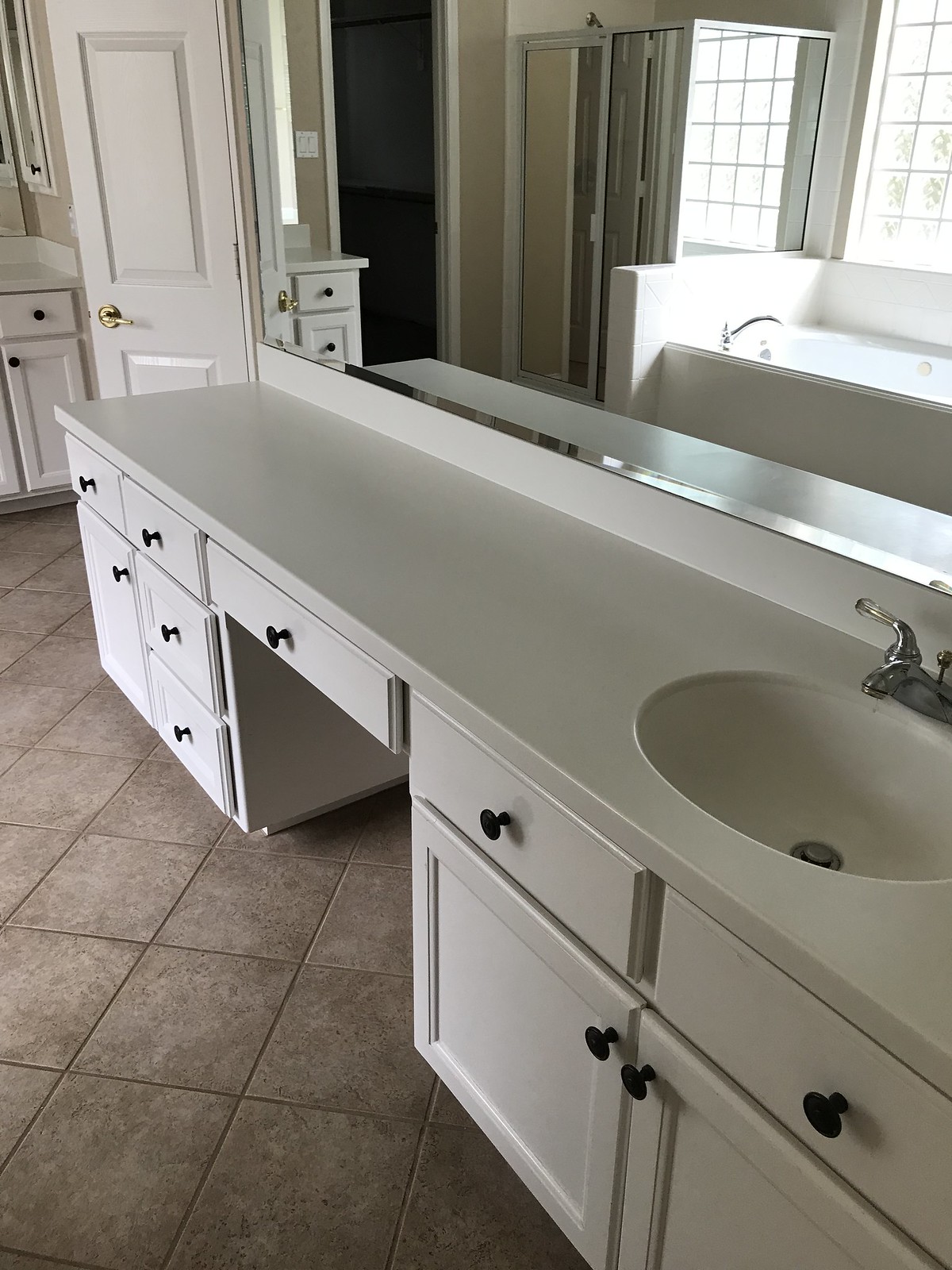The image depicts a spacious, luxurious bathroom with a meticulously designed layout. In the foreground, an elegant sink is inset into a long, extensive countertop. This countertop is supported by a series of cabinetry which includes one, two, or possibly five drawers lined just under the lip of the countertop, accompanied by another set of five varying-sized cabinets positioned below. The cabinetry features round knobs and is colored in a light tan hue, harmonizing with the brown tiled floor beneath. There is an inset section within the cabinetry potentially designed for seating, ideal for personal grooming, although it currently lacks a chair.

In the background, matching cabinetry and a similarly-colored door can be seen, complemented by a grand mirror that stretches across the wall, reflecting a lavish bathtub area. This tub, encased by walls extending approximately two feet above its rim, sits beside a large window with multiple panes, through which abundant natural light filters, illuminating greenery outside. The mirror also provides a glimpse of what appears to be the entrance to a walk-in closet on the opposite side of the room, enhancing the sense of space and luxury in this well-appointed bathroom.